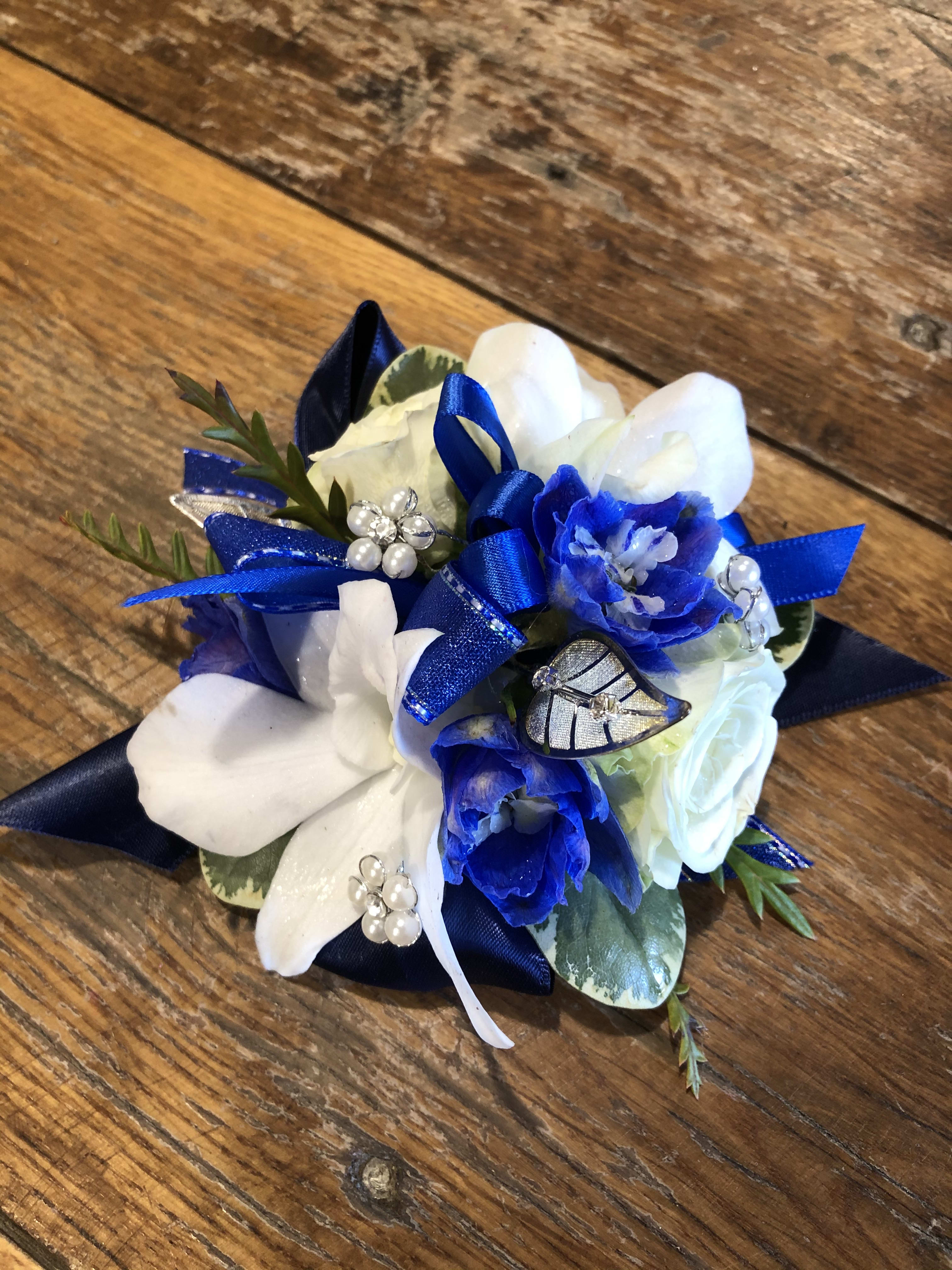This detailed photograph in a portrait layout showcases a beautifully crafted corsage or wedding bouquet, prominently featuring white roses paired with striking blue tulips. Adorned with blue ribbons and intricate pearl-like flowers, each with rhinestones or cubic zirconia in their centers, the bouquet exudes elegance and sophistication. The arrangement includes artificial silver and black leaves, some decorated with small gemstones, and hints of green foliage, adding depth and variety to the composition. The bouquet rests on a worn wooden surface, possibly a table or floor, with visible wood grain patterns providing a textured backdrop. The image focuses solely on the bouquet, highlighting its intricate design and refined details, with no text or people present.